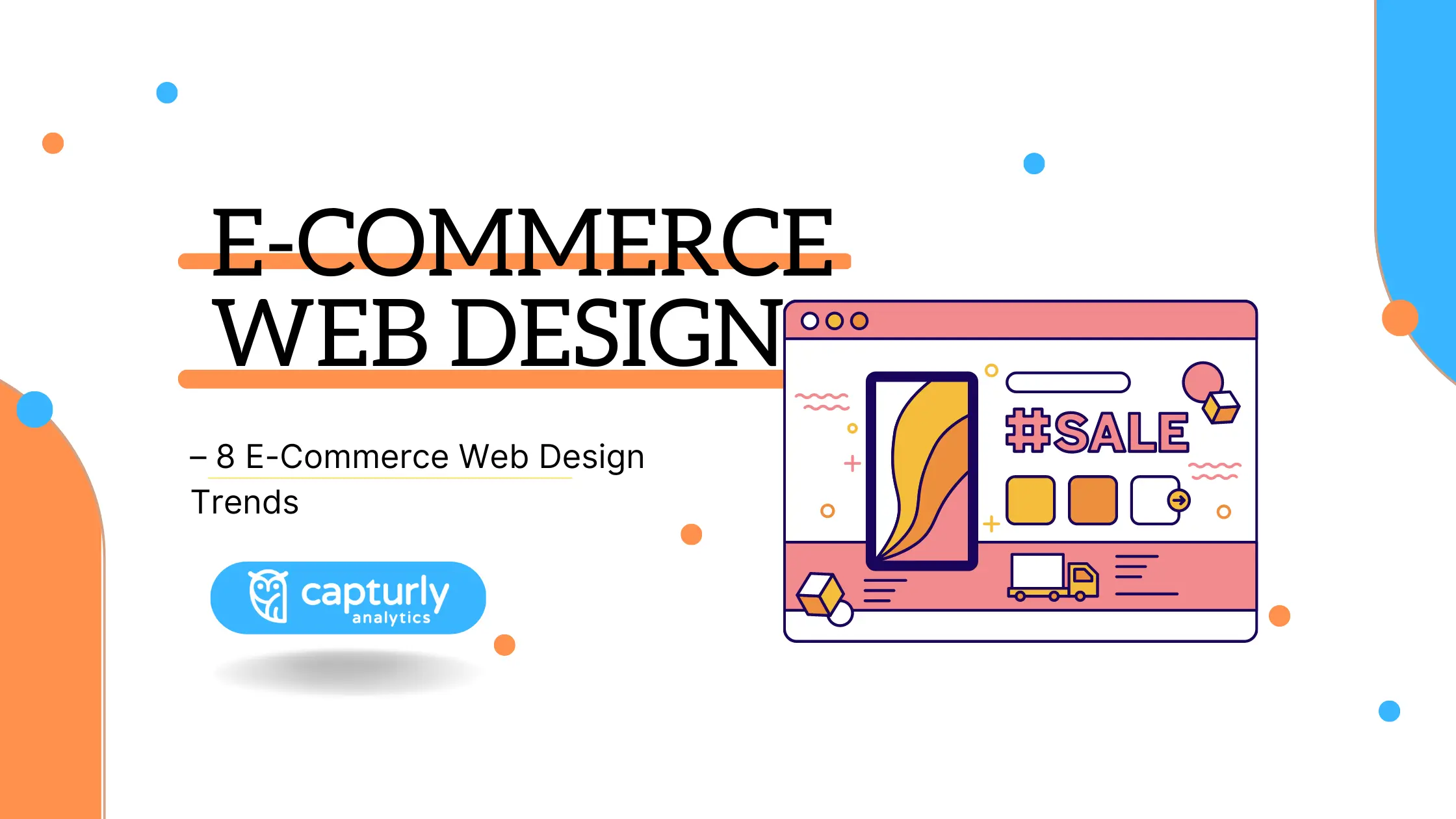This detailed advertisement showcases the latest e-commerce web design trends. It features a clean white background with the prominent black text "e-commerce web design" underlined by striking orange lines. The subheading reads “8 e-commerce web design trends.” Below this text, the logo for Capturely Analytics is displayed in an elongated blue capsule, containing a white owl clip art and white font. On the right side of the advertisement, there is a supplementary card highlighting a sale. This card includes a coral stripe on the top and bottom with a white center decorated by orange, pink, and darker orange wave-like symbols and a square that reads "#sale." The design also incorporates small orange and blue dots scattered throughout, alongside distinctive knife-shaped symbols in blue and orange.